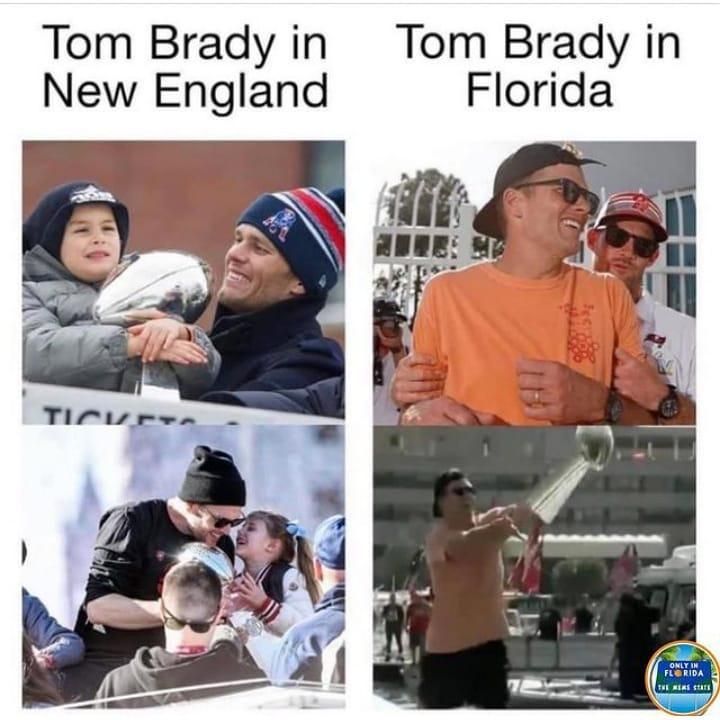A meme of Tom Brady highlights his contrasting lifestyles in New England and Florida through four distinct photos. The left side, titled "Tom Brady in New England," features two images set during the cold winter months. The top photo displays Brady with a child, both bundled up in winter attire, as they share a moment holding the Lombardi Trophy. Tom sports a blue, white, and red New England Patriots beanie and smiles lovingly at the child wrapped in a puffy gray jacket and blue hat. The bottom photo on the left shows a similar scene with Brady, wearing a black beanie and glasses, surrounded by people as he holds his daughter, who joyously clutches the trophy.

On the right side, under the heading "Tom Brady in Florida," the photos capture a starkly different, warmer vibe. The top image shows Brady in an orange short-sleeved shirt and a backwards black cap, playfully laughing as someone in a red baseball cap and white shirt guides him from behind. Below, Brady is seen in a light orange shirt, seemingly tossing the Lombardi Trophy from one boat to another, encapsulating the carefree, exuberant spirit of Florida. The bottom right corner of the meme is marked with the phrase "only in Florida" in white letters on a blue rectangle, emphasizing the state's reputation for unique and unpredictable happenings.